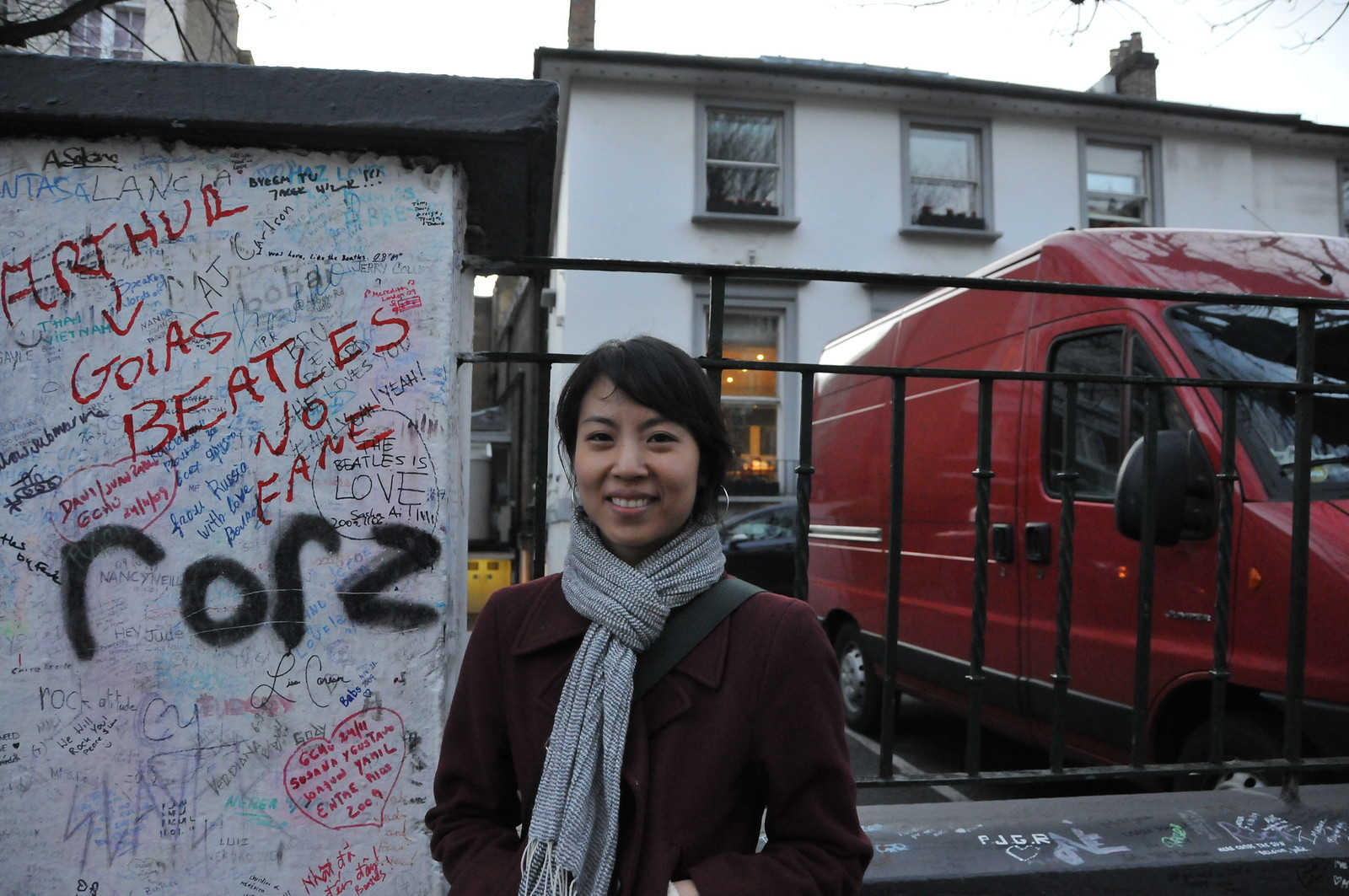In this photo, a smiling Asian woman with black hair stands outdoors in a European location during the fall. She is wearing a dark reddish-maroon coat and a gray scarf. Behind her, a white wall is covered in various colors of handwritten graffiti. To her left, which is the viewer's right, a red cargo van is parked. The building she stands in front of is white with a dark roof, and it features at least four windows reflecting the overcast, gray sky, and nearby trees.